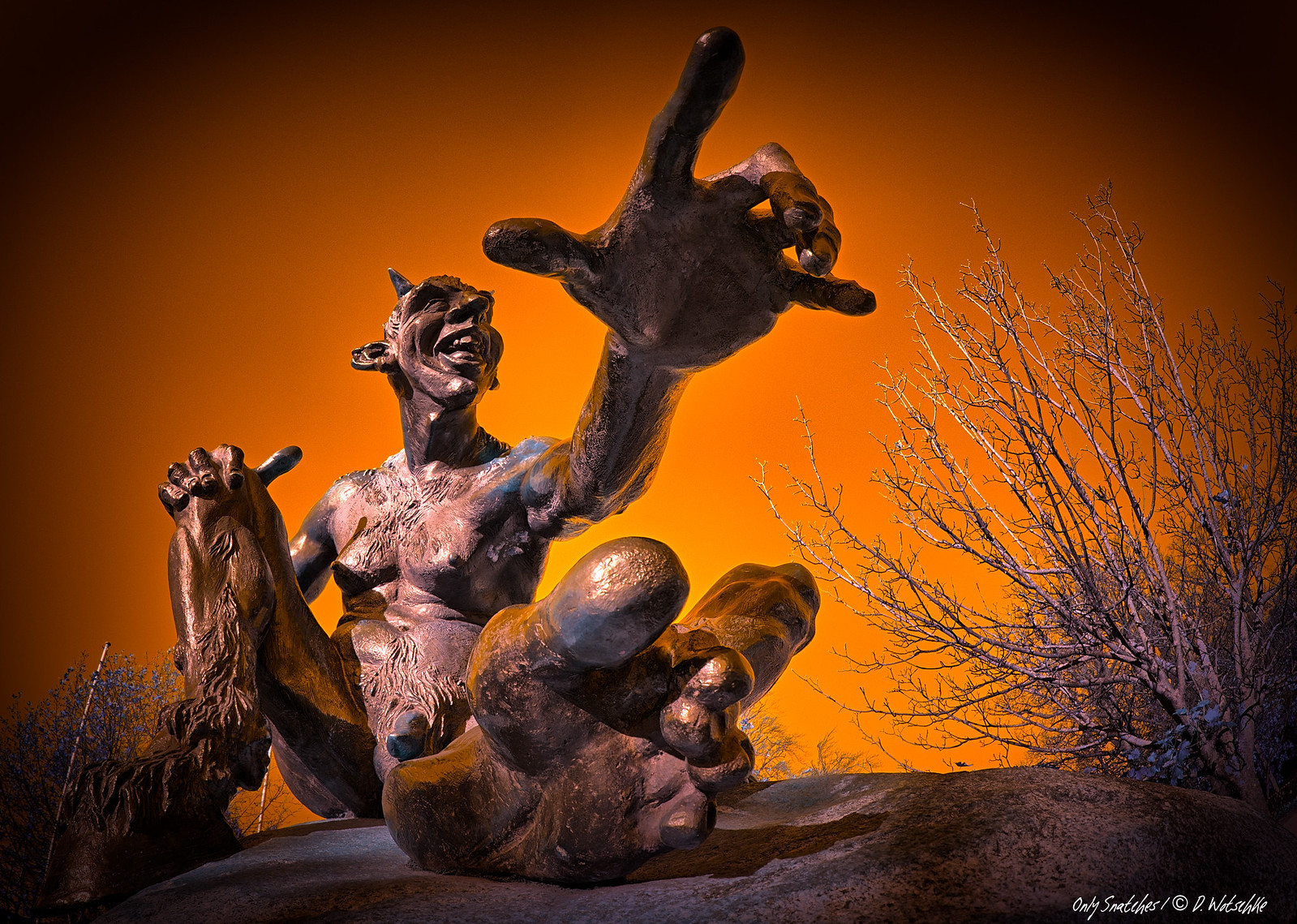The image showcases an intricately detailed sculpture of a gargoyle-like creature, centrally positioned on what appears to be a rocky surface. The creature, with its nude, flabby yet skinny physique, is seated with one leg extended towards the viewer, exposing the bottom of its oversized foot, illuminated by a glare off its brown toe. The sculpture's body exhibits a light purple hue with a hairy chest, thick pubic hair, and dense leg hair particularly noticeable towards the bottom. Its left leg is bent with the foot flat on the ground and a hand resting on the knee. The creature’s other arm is outstretched, with a finger pointing up and slightly to the left, guiding the eye towards its head. The head is adorned with large ears, a prominent nose, partially visible horns, and an open-mouthed smile. Behind the statue, a vivid orange background gradient fades into black, enhancing the dramatic aura of the piece and suggesting an indoor display. Flanking the sculpture are lifeless, bush-like plants tinged with purple at their bases. An artist's signature at the bottom right corner reads "Only Snatches Copyright. D. Welshild," adding a personal touch to the exhibition.